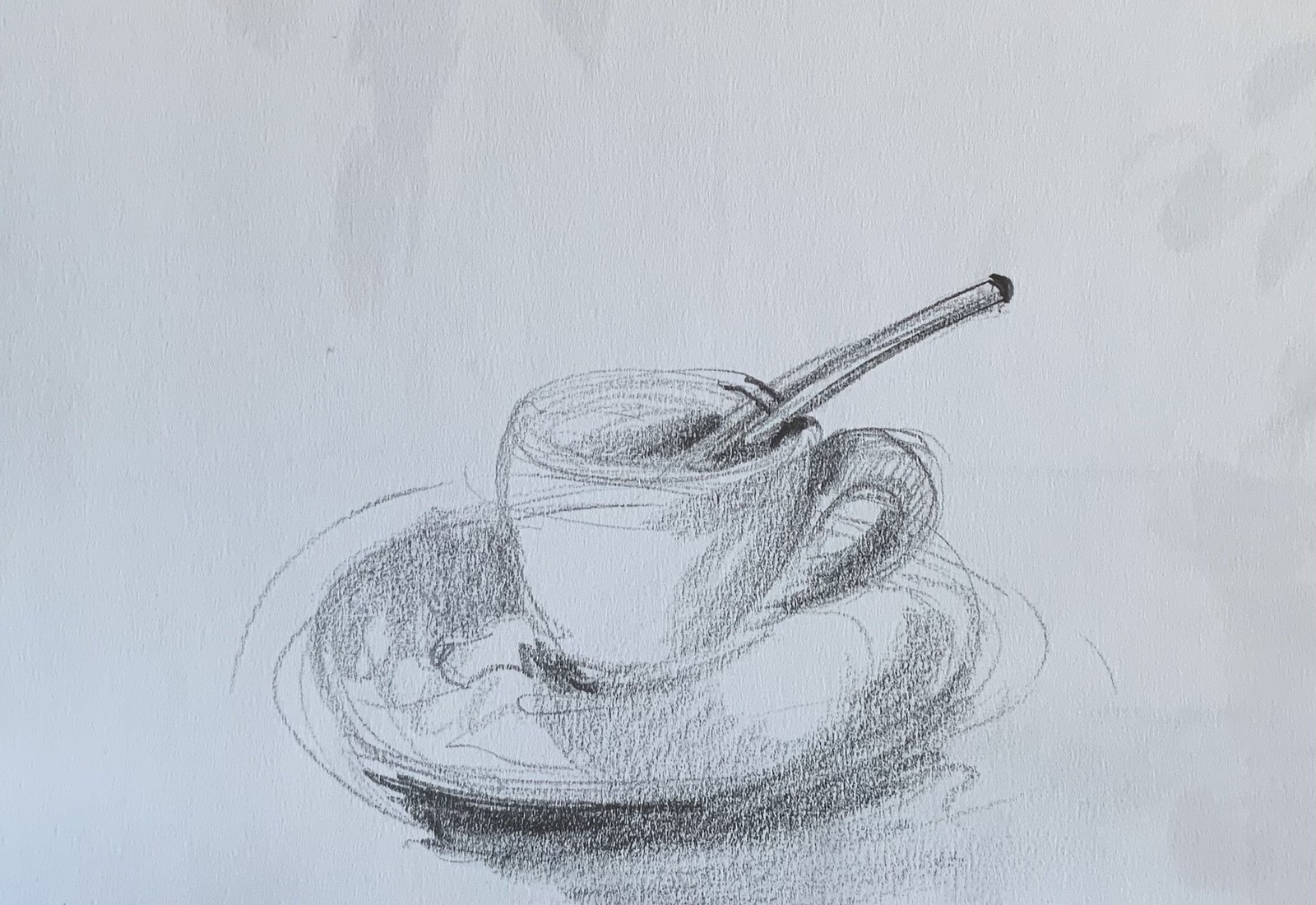This detailed pen and pencil drawing depicts a coffee cup or teacup resting on a saucer. The artwork employs intricate shading techniques to create depth and realism. Shadows extend from various points on the paper, with notable dark areas towards the left, and the top and bottom right corners. The saucer is rendered with multiple concentric circles and varies in shading intensity, becoming darker in certain sections. The teacup itself features a handle that is more heavily shaded, indicating its three-dimensional form. Inside the cup, there's intricate shading, illustrated by circular scribbles that give a textured appearance. Emerging from the cup is the handle of a spoon, suggesting it is placed inside. Below the saucer, a prominent shadow extends predominantly to the left, darkening significantly before gradually lightening as it reaches the edge of the paper.